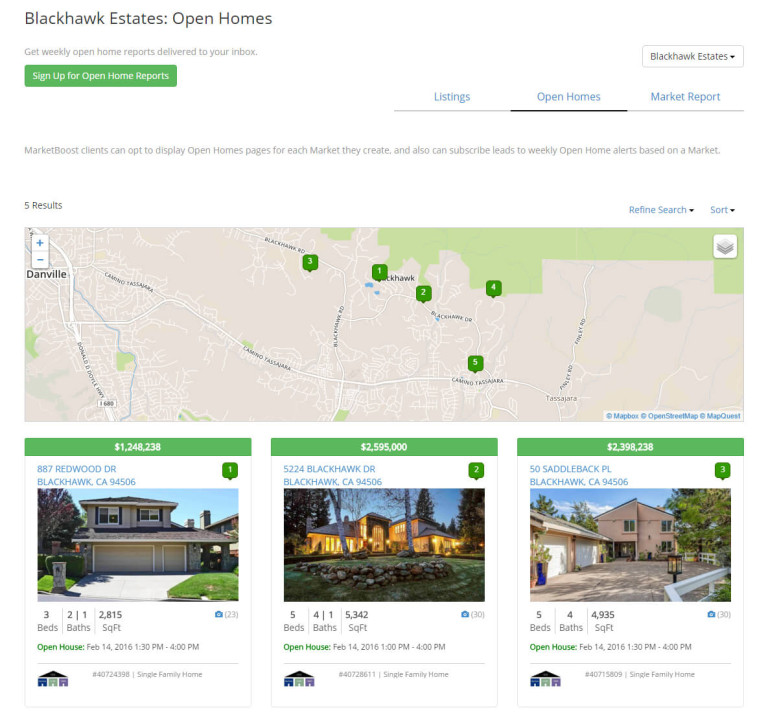The image displays a webpage from Black Hawk Estates, specifically from a section titled "Open Homes." At the top, a banner reads, "Get weekly open home reports delivered to your inbox," accompanied by an invitation to sign up for these reports. To the right, there is a Black Hawk Estates drop-down menu for easy navigation. Another menu with blue hyperlinks includes options labeled "Listings," "Open Homes," and "Market Report." 

Below, a gray line stretches horizontally across the page, beneath which a black line highlights the currently selected "Open Homes" tab. A prominent green button labeled "Sign up for open home reports" is also present. Further down, there is text explaining that Market Boost clients have the option to display open home pages specific to each market they create and can subscribe leads to weekly open home alerts accordingly.

The page includes a map dotted with green speech bubble pins, numbered one through five, indicating properties that are currently for sale. At the page's bottom, three listed properties are featured, each with an image, pricing information, the number of bedrooms and bathrooms, and additional property details.